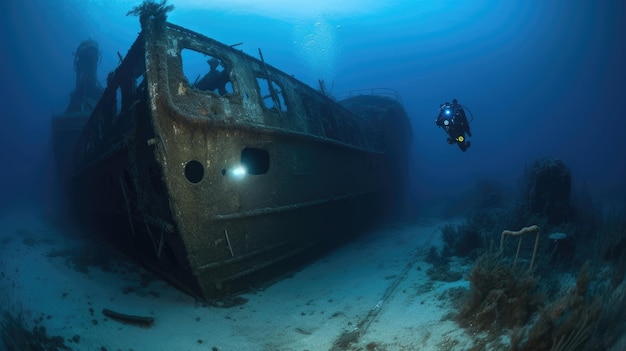This underwater photograph reveals a well-preserved scene of a sunken ship resting on a sandy ocean floor, interspersed with algae and scrub-like plants. The sunken vessel, likely from a bygone war, shows significant wear, with its rusted brown hull remaining largely intact despite the absence of its wheelhouse, mast, and other top structures. Noteworthy features include an open window near the top, a circular window, and a rectangular window lower on the hull. To the right of the ship, a diver in a heavy black scuba outfit, equipped with tanks and headlamp, prepares to explore the wreckage. The ambient light filters through the water, creating a gradient from light to dark blue, enhancing the haunting beauty of the scene. The diver’s presence, with an additional flashlight in hand, highlights the scale and mystery of the submerged relic.